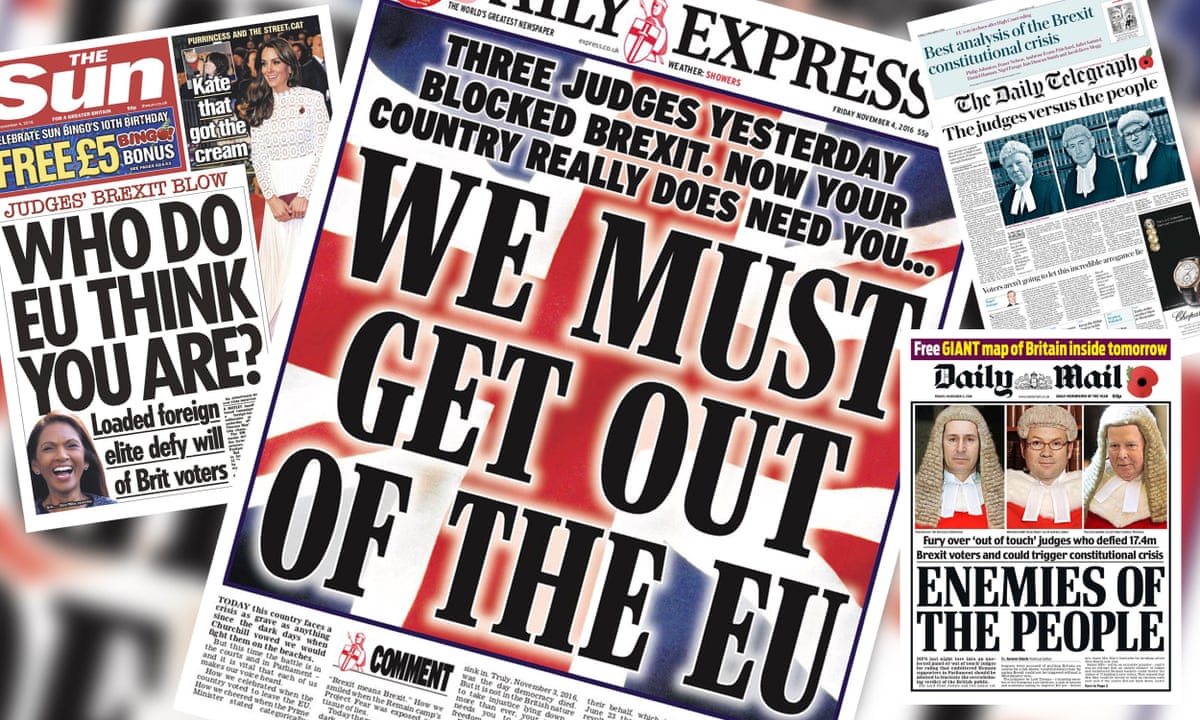The image is a detailed collage of four prominent British tabloid covers, each contributing to a narrative surrounding the Brexit controversy. Central to the composition is the front page of the Daily Express, highlighted in bold colors of red, white, and blue, declaring "Three Judges Yesterday Blocked Brexit. Now your country really does need you... We must get out of the EU." To the left, the smaller yet conspicuous cover of The Sun features headlines like "Judges Brexit Blow" and "Who Do EU Think You Are?" accompanied by an image of Kate Middleton with the caption "Kate that got the cream." On the top right, the Daily Telegraph's headline, "The Judges vs The People," is paired with images of three judges in traditional British judicial attire. Below it, the Daily Mail intensifies the rhetoric with the headline "Enemies of the People" and features color photos of the same three judges, denouncing their decision by highlighting "Fury over out-of-touch judges who defied 17.4 million Brexit voters and could trigger constitutional crisis." The background of the collage is filled with blurred, indistinct images of other newspapers, giving the entire scene an abstract and chaotic ambiance, underscoring the frenzied media reaction to Brexit.